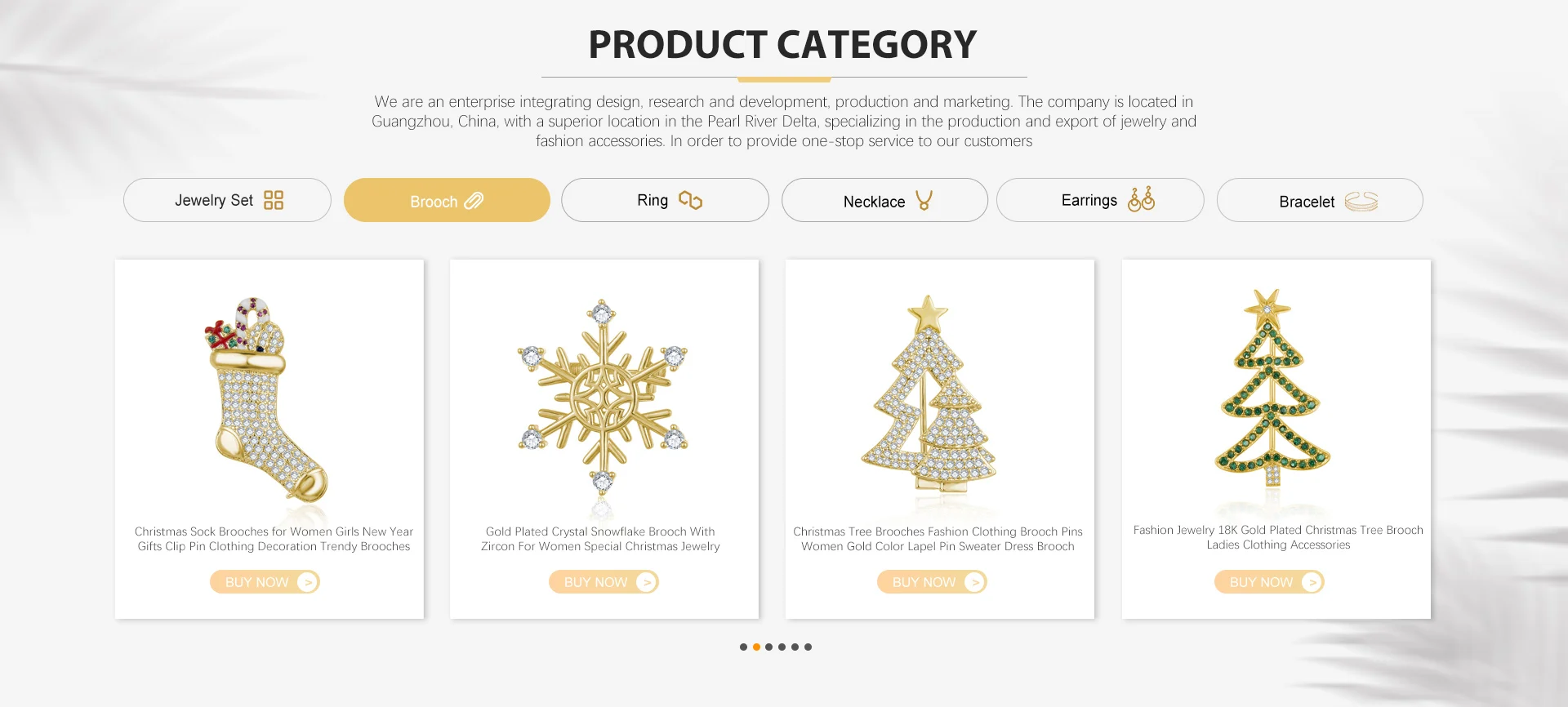A screen capture of a product category page on a website with a light gray background. The top center features the heading "Product Category" in bold black lettering. Below it, a tagline reads, "We are an enterprise integrating design, research and development, production, and marketing." The company is based in Gansu, China, strategically located in the Pearl River Delta, and specializes in the production and export of jewelry and fashion accessories. The page aims to offer a one-stop service for customers with a series of clickable category buttons beneath the tagline.

Starting from the left, the buttons list "Jewelry Set," followed by a mustard yellow-highlighted "Brooch," and then "Rings," "Necklace," "Earrings," and finally "Bracelet." Below these buttons are four featured images. The first image on the left shows a jeweled Christmas stocking adorned with gemstone-colored stones, including motifs of a gift and a candy cane. Next is a gold and cubic zirconium snowflake. The third image displays a gold Christmas tree inlaid with cubic zirconium and topped with a gold star. The final image features an 18-karat gold-plated arrangement of green stones topped with a gold star.

At the bottom, a navigation aid consists of six dots. The second dot is highlighted in orange, in contrast to the others which are black, indicating the current position in the image carousel.